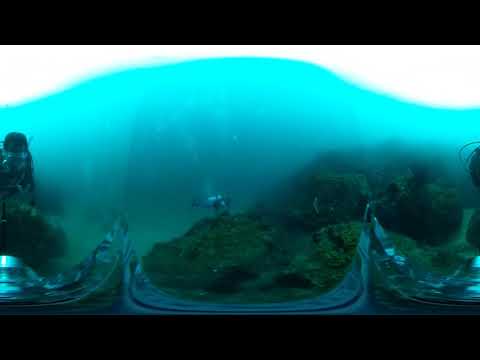The image captures a panoramic, 360-degree underwater scene, characterized by its grainy and distorted quality. Dominated by various shades of blue representing the turquoise water, the photo appears to have been taken by another scuba diver. Centrally located towards the left, there is a distant scuba diver lying on their belly, pointing to the right, and equipped with a white oxygen tank. The diver seems to be interacting with a large, green, moss-covered underwater formation. Farther in the backdrop, another diver is faintly visible on the left-hand side. The seafloor is scattered with sea rocks, adding texture to the scene. The image shows a gradient of light, with brighter, natural illumination at the top transitioning into darker depths. The bottom part of the image includes a warped and distorted reflection, possibly from a glass surface, further adding to the surreal and fragmented nature of the underwater panorama.